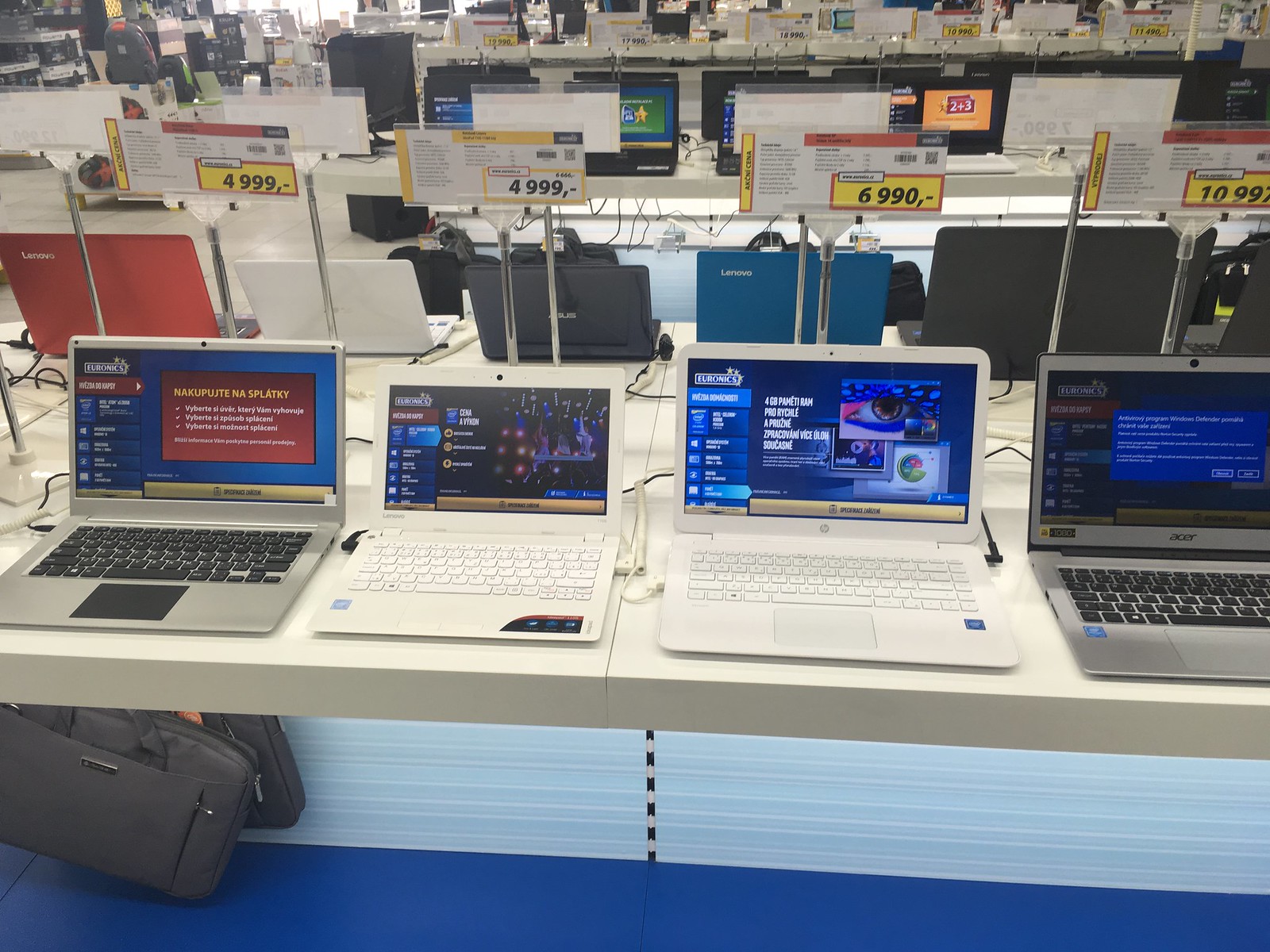This photograph, taken in an electronics retail store outside the United States, showcases a display of multiple laptops. Positioned on a sleek white island table with blue accents and carpet, four featured laptops in various colors—silver, white, and gray—are prominently lined up. Each laptop screen displays different content, with one notable screen showing a blue background with a big red box, another with a mysterious background image, a third displaying multiple open windows, and the fourth showing an error message in a blue box. The majority of the laptops seem to operate on Windows, and languages on the screens suggest non-English settings.

Beneath the table, computer bags are available for purchase, and behind this main display, additional rows of laptops are visible, indicating the extensive selection available in the store. Yellow price tags are prominently displayed above the laptops, with prices such as $4,999, $6,990, and $10,997 marked in large black writing. The laptops exhibited include familiar global brands, adding to the variety. This detailed scene illustrates the bustling environment of a well-stocked electronic retail shop filled with modern and diverse tech options.